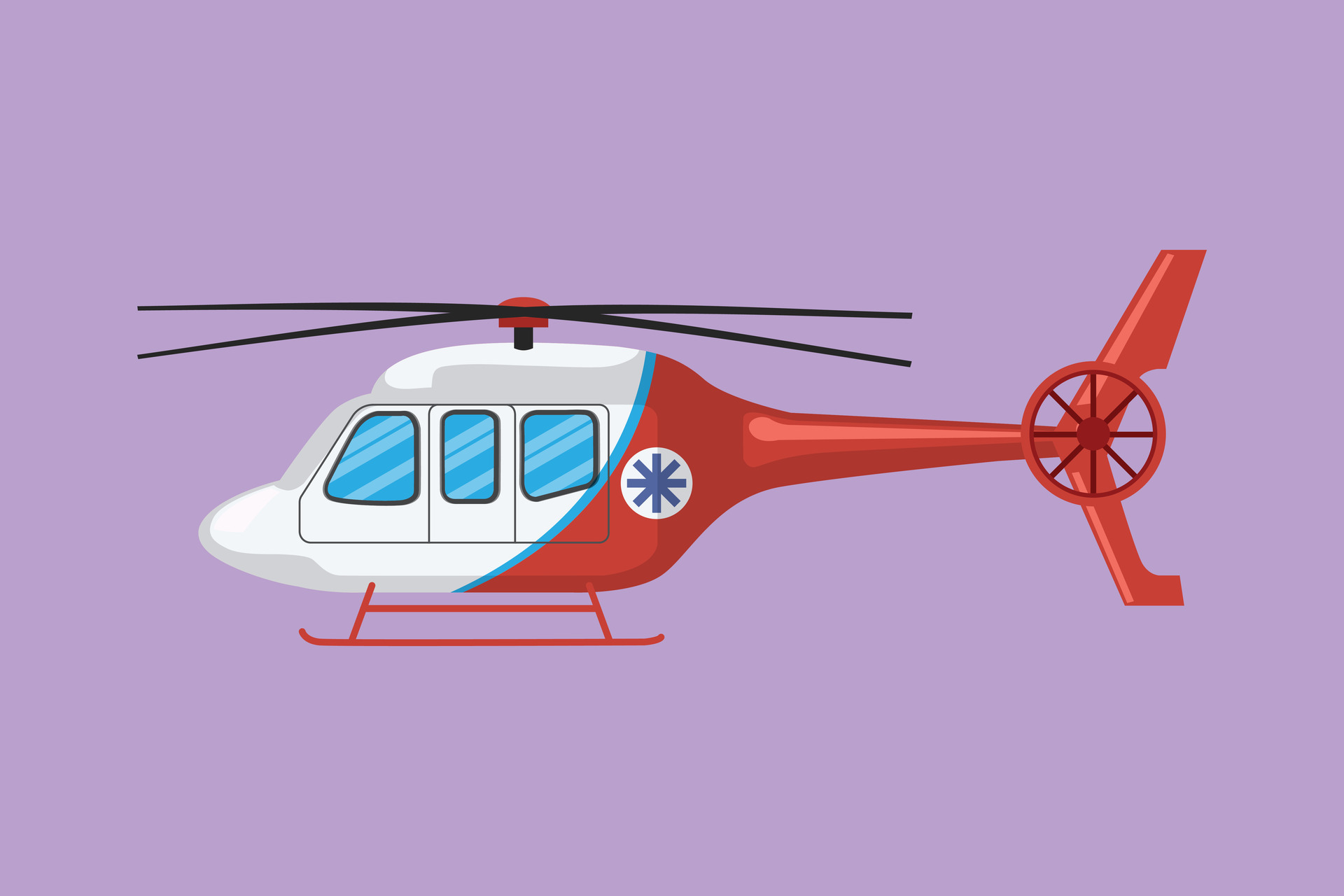This is a detailed illustration of a helicopter set against a light purple background. The helicopter, viewed from the side and centered in the image, features distinct sections and components. The front half of the helicopter is predominantly white, accented by a narrow blue stripe. It showcases three windows shaded in blue, outlined in black, representing blue glass. The back half of the helicopter is red, distinguished by a white circle featuring a blue asterisk or starburst logo. The rotor blades, both on the top and the landing skids, are black. The top rotor blades are attached via a red knob connected by a black dowel. A simple wheel with spokes is located at the very back. Overall, the drawing presents a clean, straightforward depiction of the helicopter’s structure and design elements.